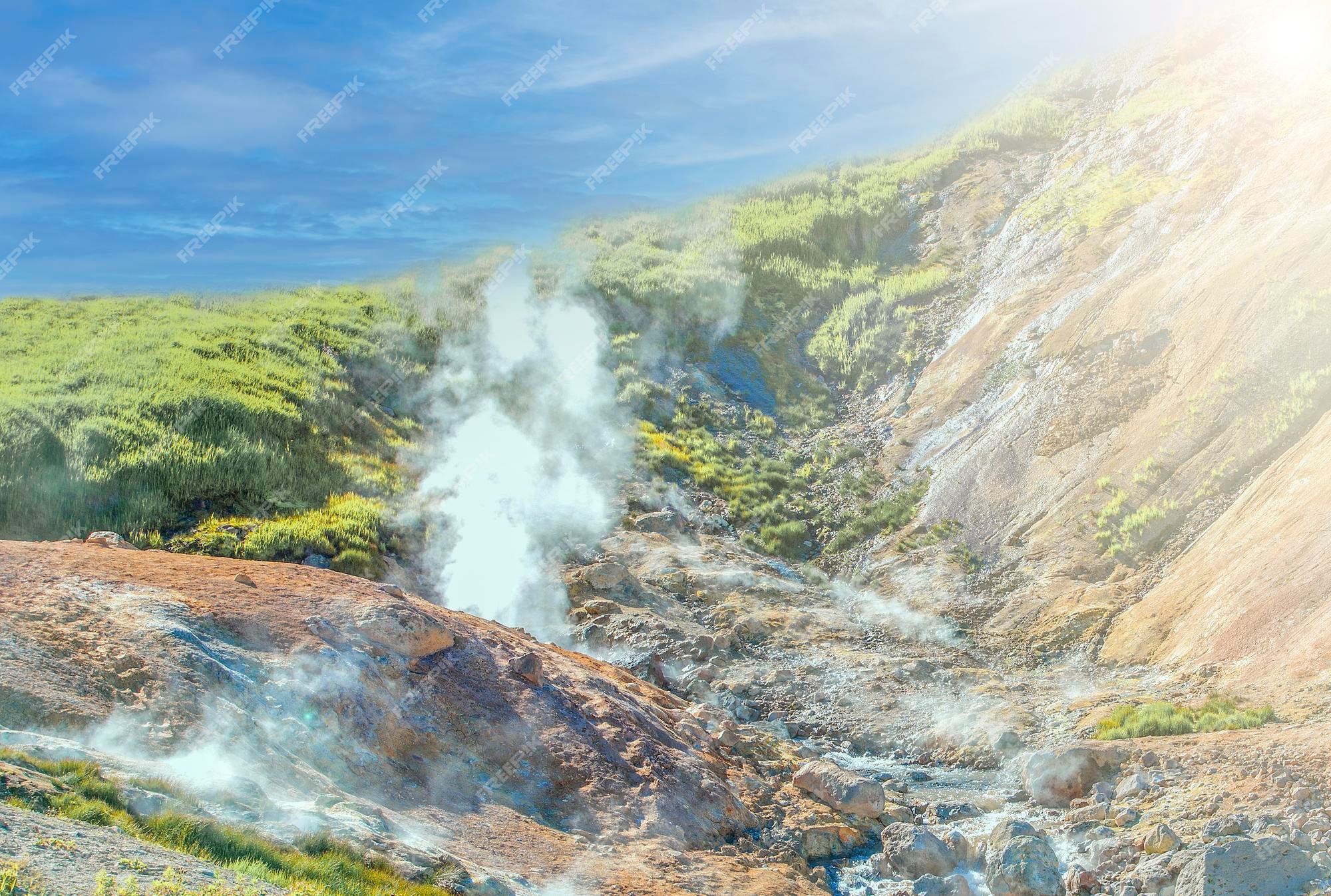This photograph captures a stunning outdoor scene of hot springs nestled within a valley. The central focus is a thermal spring with steam rising from the water and rocks, suggesting geothermal activity. Water flows from the lower right corner towards the center, adding dynamic movement to the composition. To the left, there’s a large rock with water both above and below it, accompanied by patches of green grass or possibly algae. The right side features a prominent rocky cliff extending from the upper right, framing the scene with rugged terrain. In the backdrop, a grassy area extends towards a bright blue sky adorned with streaks of white clouds. The foreground on the left side also has an elevated rocky section, creating a natural depression in the landscape. The mood is slightly disturbed by a semi-transparent white watermark with the text "free pics" diagonally spread across the image. The overall color palette includes blue skies, white clouds and steam, green grasses, and red-brown rocks, contributing to the vibrant and earthy feel of the photograph.